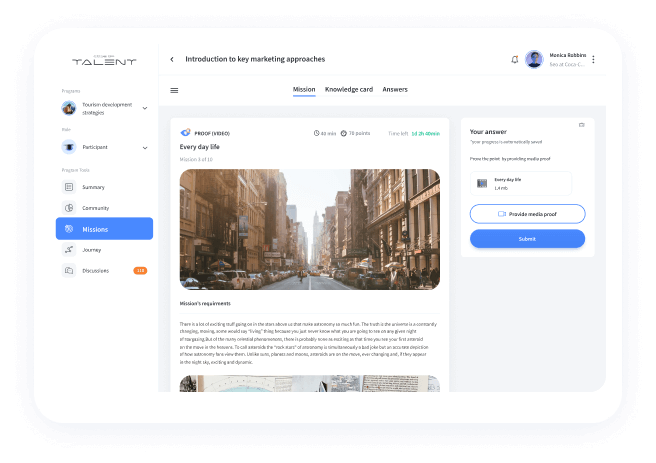The image features a predominantly white upper section, transitioning to various shades of blue on the left side, though the details remain blurry. Below this, the word "talent" appears in black, accompanied by other indistinct words. Two circles, possibly profile pictures, are visible; one is a mix of blue and white, while the other is blue and black with the word "participant" nearby. Below these elements, phrases such as "tools," "summary," and "community" are written in black, leading to the word "missions" in white that stands out against a blue highlight. The term "journey" follows in black text, concluding with an unidentifiable word next to an orange oval containing blurred white numbers, possibly "118," "115," or "110."

Further down, the caption "introduction to key marketing approaches" is written in black, followed by three black horizontal lines and an underlined "mission" in periwinkle. Additional text includes "knowledge card" and "answers" in black. The background features a gray area with a white rectangular border, containing the phrases "everyday life" and "mission," possibly indicating "one of 10." The scene depicts brownstone buildings on either side of a street with parked cars and an abundance of blurry words beneath.